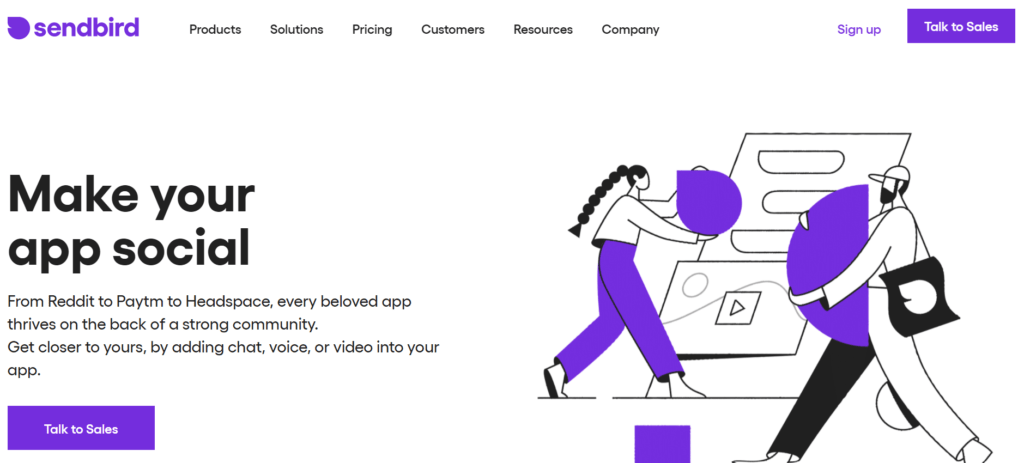This image is a cropped screenshot of the Sendbird homepage. At the top left, the vibrant purple Sendbird logo stands prominently. To its right, a navigation bar with category listings stretches across the page, featuring "Products," "Solutions," "Pricing," "Customers," "Resources," and "Company." On the far right, "Sign Up" is displayed in a small purple font. Adjacent to it, a rectangular "Talk to Sales" button stands out, inviting potential customers to reach out.

The body of the page has a clean white background. To the left, in bold black letters, the tagline "Make your app social" catches the eye. Below this, a succinct description reads: "From Reddit to Paytm to Headspace. Every beloved app thrives on the back of a strong community. Get closer to yours by adding chat, voice, or video into your app." Beneath this text, a purple "Talk to Sales" bar is prominently displayed.

To the right side of the screen, a series of clipart images depict a woman and a man, both in black and white, carrying various geometric shapes. Behind them, graphical elements of web pages provide context. The man has a bag slung over his shoulder, adorned with the Sendbird logo. This illustration adds a human touch to the otherwise technical presentation. The screenshot is wide enough to capture the top panel of the website, highlighting the essential elements of the homepage.